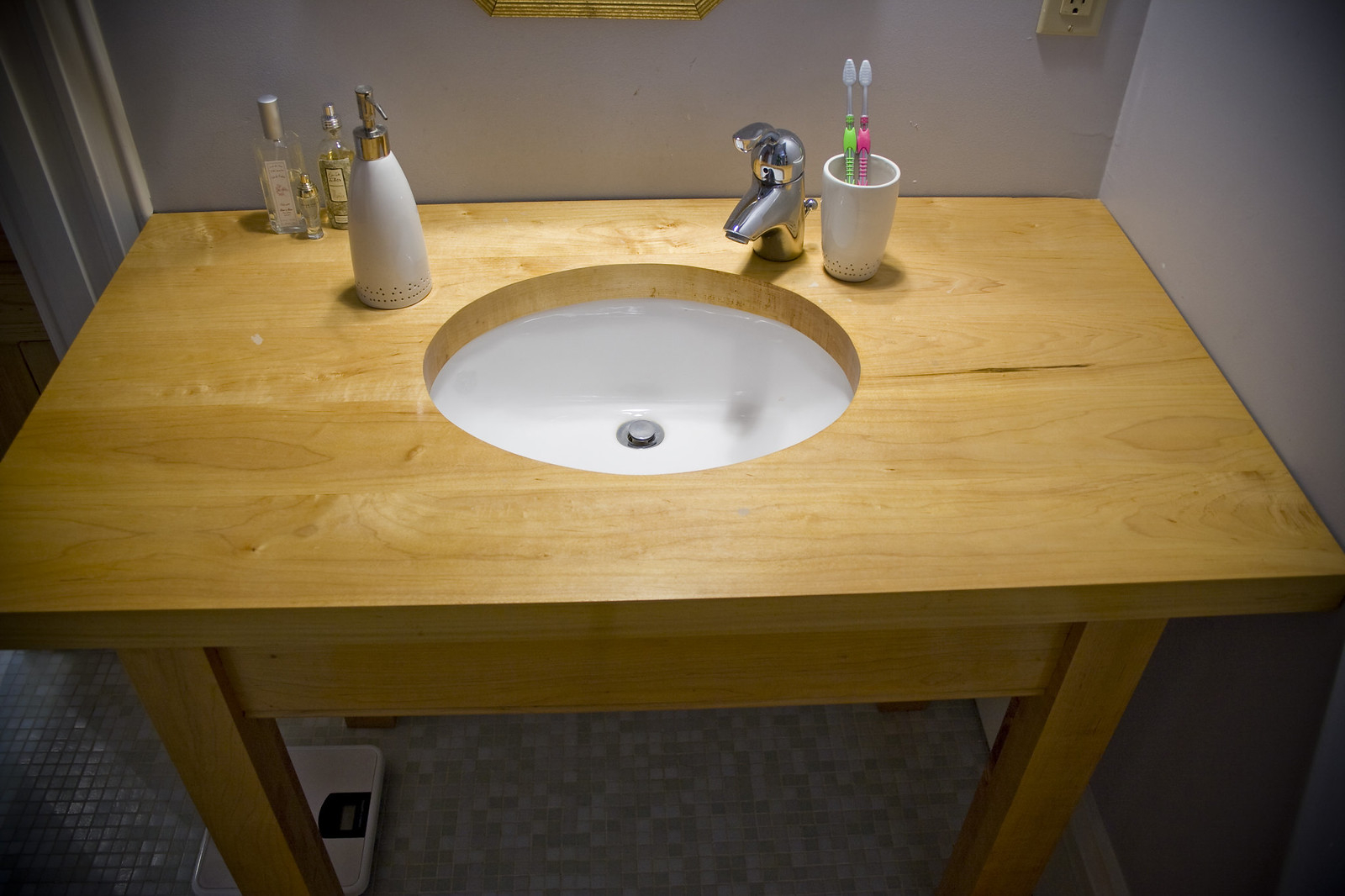This image captures a unique bathroom sink setup that integrates rustic and modern elements. The sink is embedded within a wooden tabletop, which has a precisely cut hole to accommodate a white porcelain basin. The basin features a gleaming chrome drain at its center, adding a touch of sleekness to the ensemble.

A contemporary water spigot, equipped with a single handle for adjusting water flow and temperature, is mounted on the upper right section of the wooden tabletop. To its immediate right stands a white cup holding two toothbrushes, easily distinguishable by their vibrant pink and green colors.

Positioned to the left of the basin is a white soap dispenser with a chrome pump handle, radiating a minimalist elegance. Behind the soap dispenser, three perfume or cologne bottles are neatly aligned—two larger bottles flanking one smaller bottle.

The bathroom floor is adorned with gray and white tiles, adding a subtle texture to the space, while a digital scale rests beneath the sink, ready for use. The walls are painted a calming gray, complementing the overall decor. Above the sink, a light fixture casts a direct beam, illuminating the area and highlighting the details.